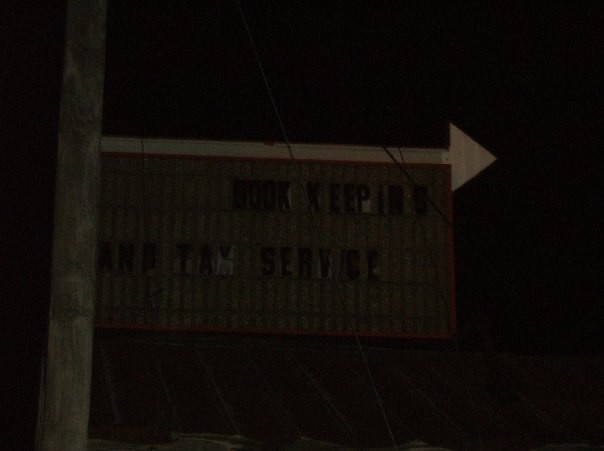This is a photograph shrouded in darkness, rendering the background nearly indistinguishable as an empty black void. Amid the inky obscurity, vague shapes resembling a distant rooftop can be discerned, characterized by their deep brown, almost black hues. Anchored in the murky foreground stands a tall wooden pole, atop which a sign is precariously visible despite the overwhelming dimness. Struggling to pierce the gloom, one can just make out a white arrow pointing to the right at the top of the sign, with the faintly readable inscription beneath it: "Bookkeeping and Tax Service." The pervasive darkness challenges any attempt to easily discern these details, enveloping the scene in a near-impenetrable shadow.